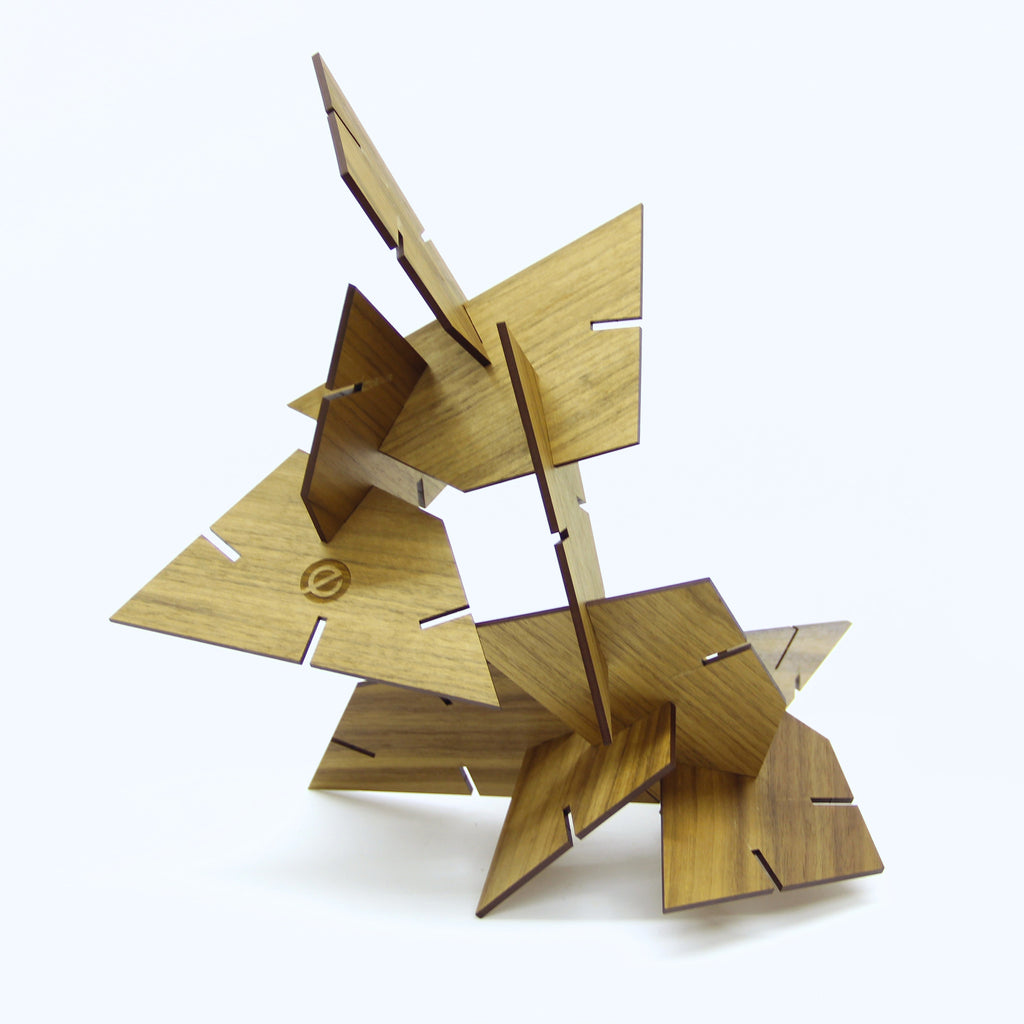This color photograph displays a complex wooden art piece that stands against a light gray, almost off-white, background. The sculpture, constructed from eleven pieces of light-colored wood, possibly walnut, is assembled using a tongue-and-groove system. Each piece of wood features four notches: one at the bottom and midpoints on each side, facilitating their interlocking formation. The individual wooden components are four-sided with an angled inward left and right side, and a flat base, tapering to an angular upward top. The structure begins with an angular base on the ground and extends vertically to form a dynamic, angular mass at the top. Notably, one piece on the front left bears an engraved lowercase 'e'. The overall design is reminiscent of a three-dimensional wooden puzzle, with variably shaped and sized pieces interlocking to create a cohesive, standing sculpture.